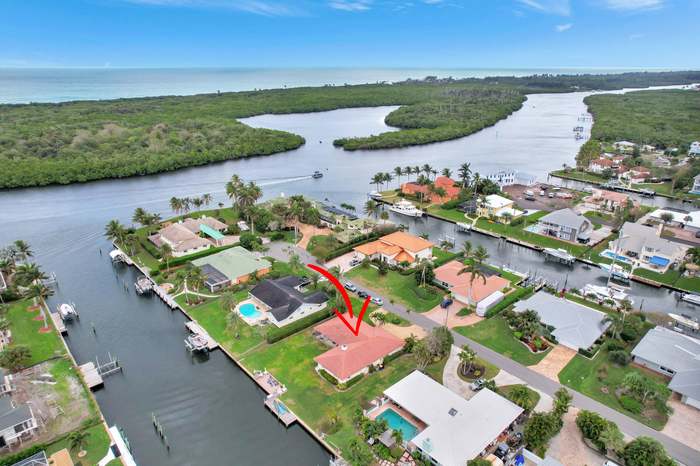This detailed aerial realty photograph captures a picturesque coastal neighborhood that appears to resemble a Florida setting, complete with homes strategically nestled along a winding river and its interconnected waterways. Central to the image is a red arrow pointing to a house with a distinctive red roof, positioned prominently in the middle of the photo. The neighborhood, composed of several clusters of homes, features three visible islands intertwined with inlets and flanked by docks and boats, accentuating its waterfront charm. On the left side of the image, a row of homes stretches alongside the water, each accompanied by individual boat docks and some with backyard pools. In the center, two additional rows of houses similarly exhibit a harmony with the water, accentuated by more docks and boats. Further sections reveal an intricate layout of little canals and rivers, interspersed with flourishing vegetation and trees that line the coastline. The background extends into the horizon, depicting marsh areas and the river that winds gracefully all the way through the picture, eventually merging with the distant expanse of the ocean beneath a serene blue sky.